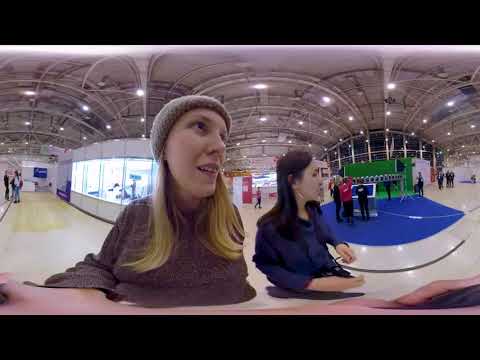The image is a panoramic photo of two women standing at a convention hall with a tall, white-painted ceiling featuring multiple bare metal support rafters and round light fixtures hanging at intervals. The woman on the left is visible from the waist up, wearing a soft, long-sleeve zip-up jacket, possibly purple or brown, with long blonde hair cascading past her shoulders. She is adorned with a gray or tan knit beanie on her head. The woman to her right is also visible from the waist up, dressed in a blue business coat and shirt, with long black hair. Both women are looking to their left with amused expressions, possibly resting their hands on an unseen counter or table.

Surrounding them are multiple exhibit booths, and several people can be seen in the background engaged in different activities, including looking at a monitor. The floor is made of white tiles, and there's a blue rug visible in the right background. The left background features a corridor with what appears to be a glass window, bordered in white, containing indeterminate items behind it and potentially an exit door. The image, taken with a 360-degree camera, shows some warping, particularly noticeable on the woman on the left, whose hands appear distorted towards the edges of the frame. The setting is suggestive of a bustling convention or demonstration event.